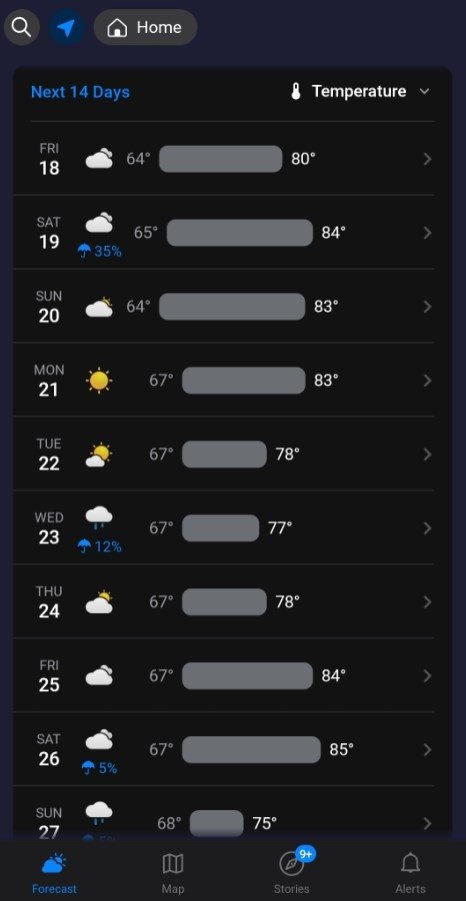The image displays a black screen interface with various weather forecast details. 

On the top left corner, there is a white magnifying glass icon representing the search function. Next to it is a blue arrow icon, followed by a white home icon. Below these icons, the text "Next 14 days" is displayed in blue. 

On the right side of the screen, the text "Temperature" is accompanied by a downward-pointing arrow. Below this, the forecast is detailed day by day:

- **Friday, 18th**: Cloudy with temperatures ranging from 64 to 80°F. 
- **Saturday, 19th**: Cloudy with a chance of rain at 35%, temperatures between 65 to 84°F.
- **Sunday, 20th**: Cloudy, temperatures ranging from 64 to 83°F.
- **Monday, 21st**: Sunny with temperatures from 67 to 83°F.
- **Tuesday, 22nd**: Partly sunny with temperatures ranging between 67 to 78°F.
- **Wednesday, 23rd**: Cloudy with a 12% chance of rain, temperatures from 67 to 77°F.
- **Thursday, 24th**: Partly cloudy, temperatures ranging between 67 to 78°F.
- **Friday, 25th**: Partly cloudy with temperatures from 67 to 84°F.
- **Saturday, 26th**: Cloudy with a 5% chance of rain, temperatures ranging from 67 to 85°F.
- **Sunday, 27th**: Rain with incomplete information on the chance of rain, temperatures from 68 to 75°F.

Each day listed includes a right-pointing arrow next to it, and a gray line separates the entries. The overall layout is designed for easy comparison of weather conditions day by day.